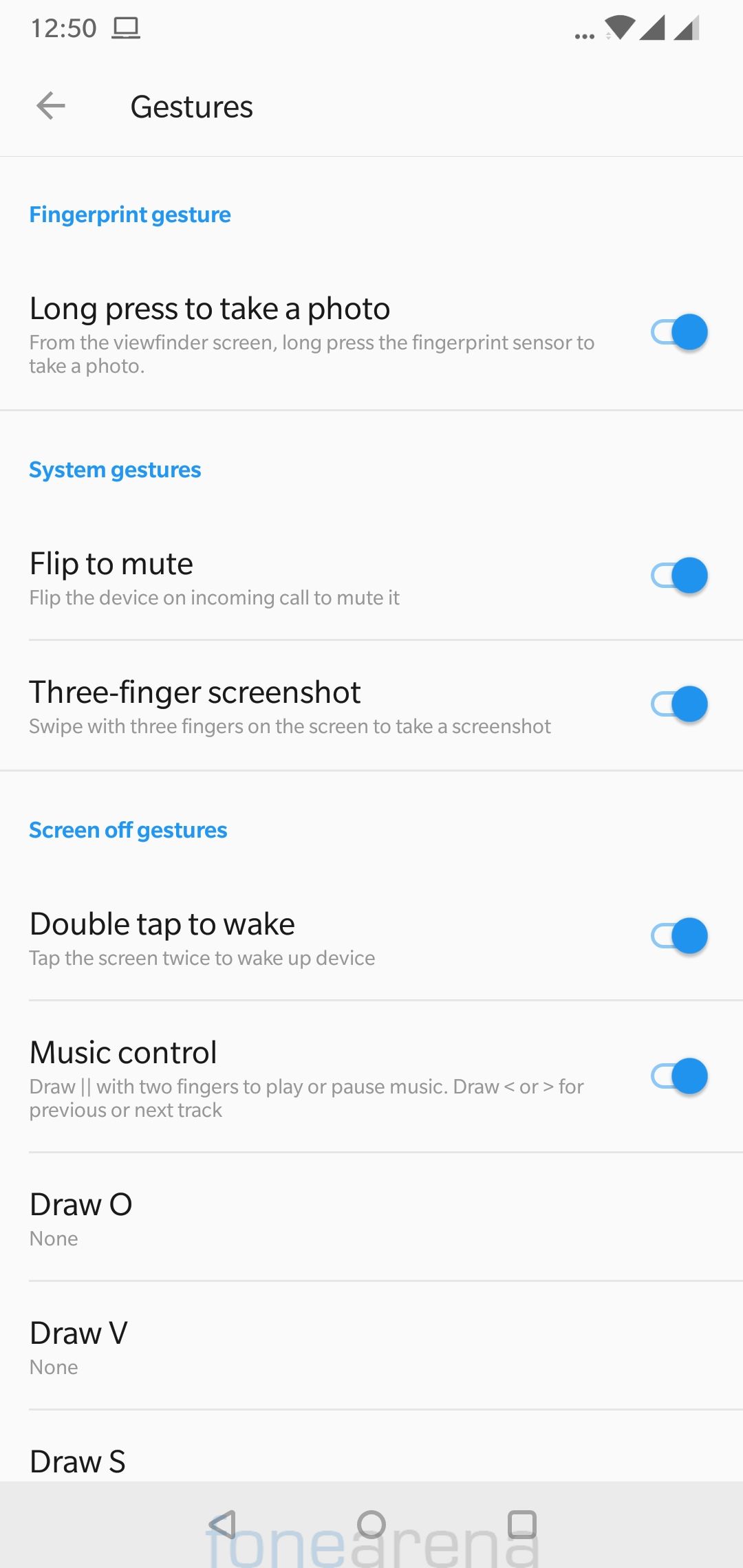The image showcases a settings menu on a device, likely within an APC (Advanced Personal Computer) interface. At the top of the screen, a clock displays the time as 12:30. Below the time, the interface is divided into several sections. 

The first section is labeled "Gestures" and features a subheading in blue text, "Fingerprint Gestures." Under this, the settings option "Long press to take a photo" is described in larger text and is enabled.

Separated by a thin gray line, the next section is "System Gestures." Here, two options are visible:
1. "Flip to mute" — Flip the device to mute incoming calls, which is enabled.
2. "Three-finger screenshot" — also enabled, but detailed in a separate category beneath the primary options.

Another category within the gestural settings showcases "Screen Off Gestures," with the following options:
- "Double-tap to wake" is enabled.
- "Music control" is enabled.
Both enabled icons are highlighted in blue.

Further down, separate columns list custom gestures:
- "Draw O" — Action is currently set to "None."
- "Draw V" — Action is also set to "None."
- "Draw S" — No action or description specified.

At the bottom of the screen, the navigation bar includes a back button, a home button, and a button for switching between apps. 

The overall design of the interface is simplistic with a white background accentuated by blue and black text and iconography. A subtle gray margin is also noticeable at the top of the screen, enhancing the minimalist aesthetic.